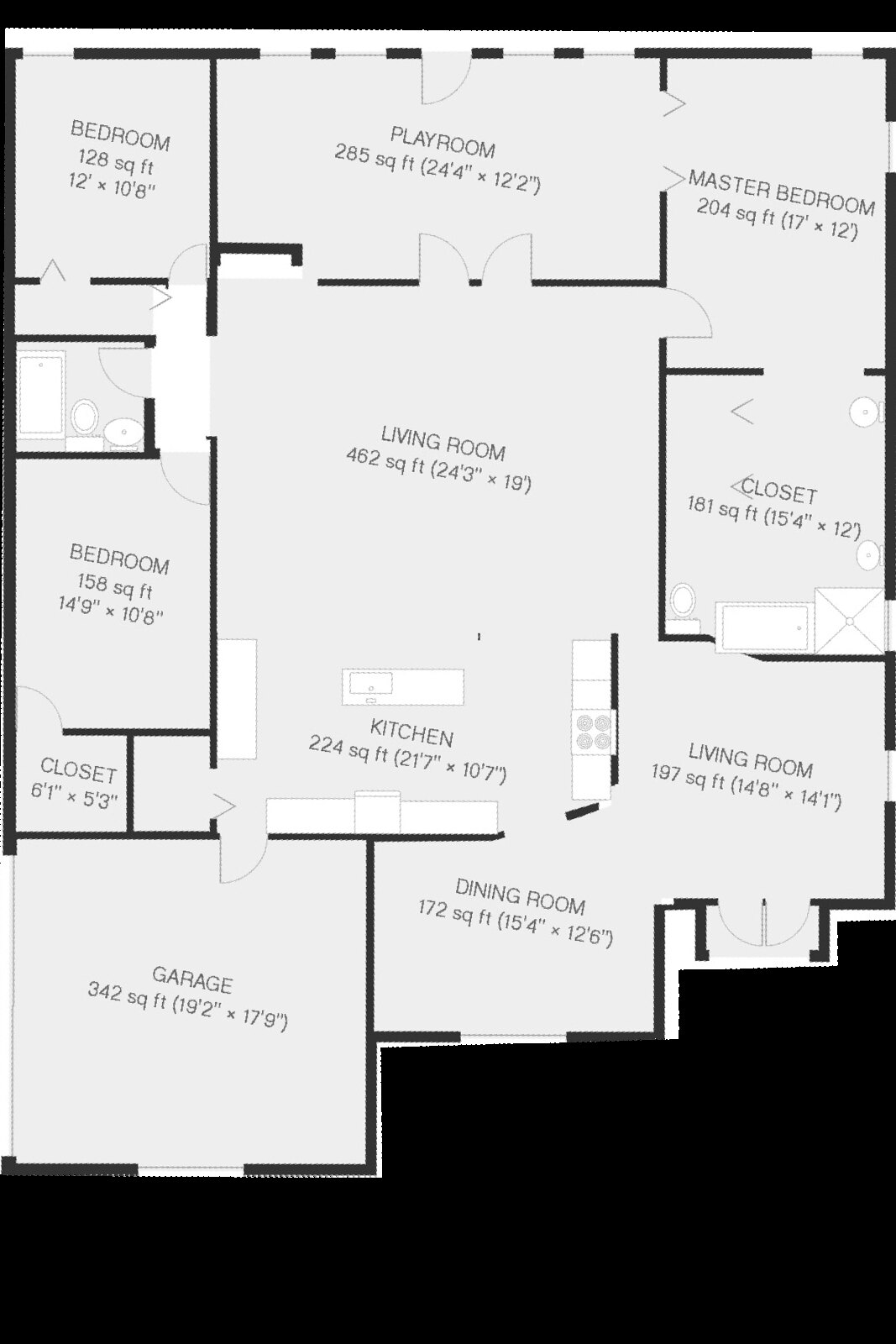The image depicts an architectural blueprint of a house floor plan, rendered in black and gray tones. The noticeable feature at the very bottom of the blueprint is a large black area, which could potentially be a basement, though it is not specifically labeled.

Starting from the left, the blueprint indicates a garage measuring 342 square feet (19 feet 2 inches by 17 feet 9 inches). Adjacent to the garage on the right, the layout opens into interconnected spaces without any wall separating them: a dining room of 172 square feet (15 feet 4 inches by 12 feet 6 inches) flows into a living room of 197 square feet (14 feet 8 inches by 14 feet 1 inch).

Continuing around the periphery, on the right-hand side, a sizable closet is detailed as having 181 square feet (15 feet 4 inches by 12 feet). This closet connects via a doorway to the master bedroom, which spans 204 square feet (17 feet by 12 feet).

On the far side of the house, a playroom occupies 285 square feet (24 feet 4 inches by 12 feet 2 inches). Adjacent to the playroom is a bedroom covering 128 square feet (12 feet by 10 feet 8 inches), though oddly, this dimension lacks parentheses. This bedroom conveniently connects to a bathroom equipped with a tub, toilet, and sink, although specific measurements for the bathroom are not provided.

Another bedroom towards the end measures 158 square feet (14 feet 9 inches by 10 feet 8 inches). Additionally, there is a small closet with dimensions of 6 feet 1 inch by 5 feet 3 inches.

In the kitchen area, the floor plan indicates various features including a countertop, an island, several counters, and a stove. The extensive closet on the right also features another bathroom complete with a toilet and bathtub, alongside an unidentified component.

The blueprint is marked with black writing on a gray background, supplemented by the conspicuous black area at the bottom that might denote a basement. This comprehensive depiction provides a detailed spatial understanding of the house's layout, emphasizing the arrangement and specific dimensions of each room.